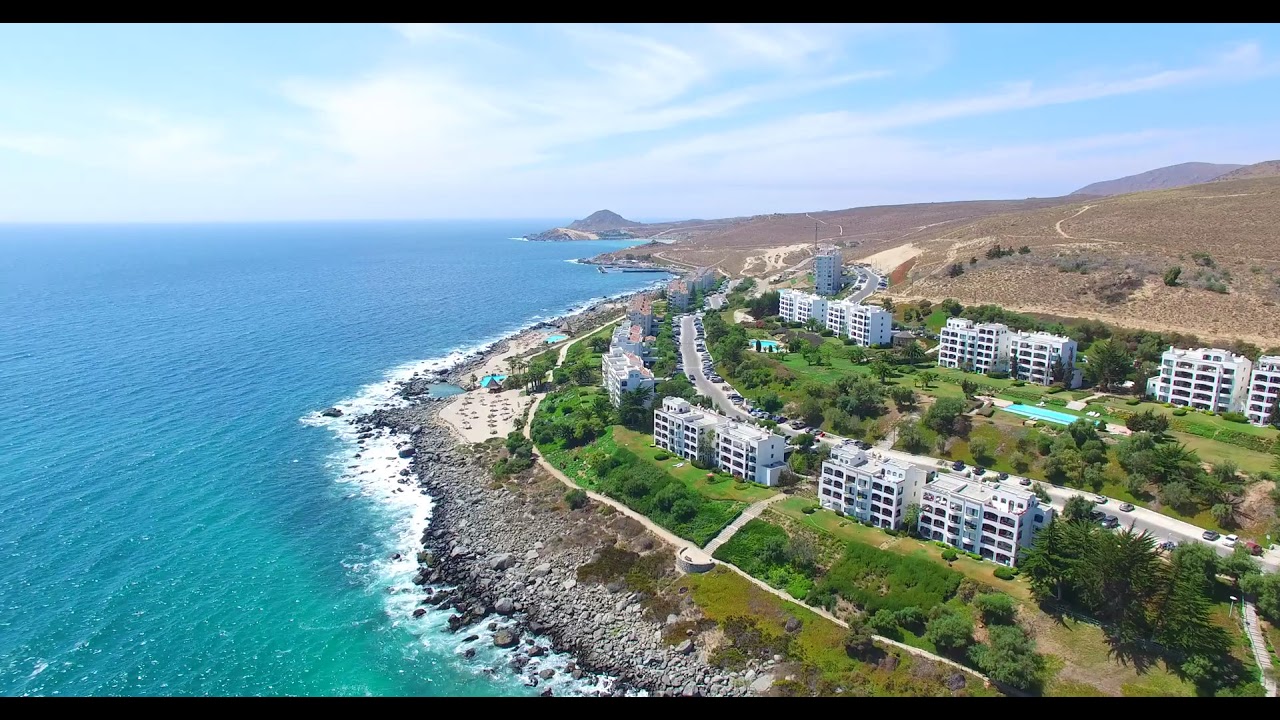The image is a detailed aerial photograph of a coastal community taken from a drone, set against a black background with horizontal strips across the top and bottom. It captures a vibrant, sunlit day at Seaside Village, possibly a resort area. The aqua blue ocean, located on the left side, transitions into frothy white waves as it meets a curved, rocky shoreline, creating a picturesque view.

The rocky beach is bordered by lush, bright green grass leading up to a row of white, multi-story condominium buildings or hotels, all similarly styled in white stucco. These buildings are likely accommodating visitors with pools adding splashes of bright blue to the scene. A path meanders from the buildings down to the coast, enhancing the picturesque quality of the landscape.

Beyond this initial line of buildings, there's a road followed by another line of identical condos or hotels, before the scenery transitions into a more gravel-like, brownish-red dirt terrain. The dirt hillside rises in the background, with a hint of a mountain range visible in the distance, further emphasizing the tranquil but vibrant beauty of this seaside sanctuary.